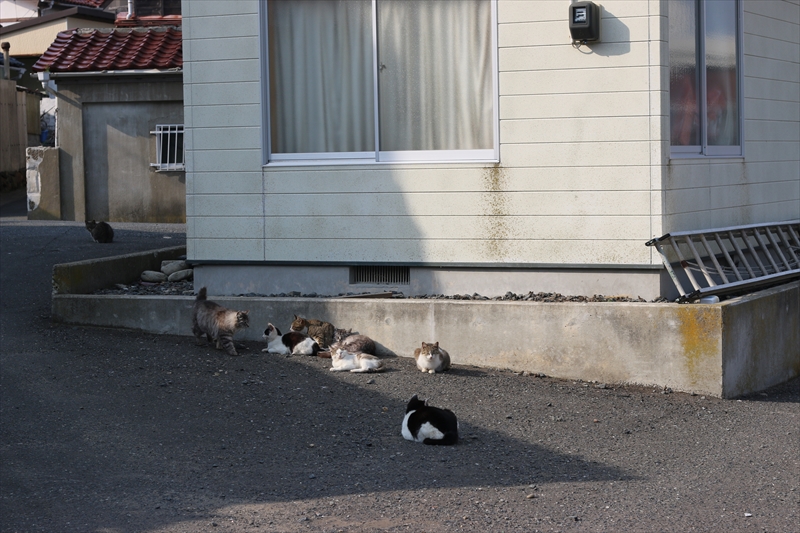In this vividly detailed image, we see a scene teeming with life and rustic charm: a cluster of about eight cats, each displaying a unique blend of colors from black and white, to gray and white, to tan and calico, lounging comfortably in front of a modest house. The cats, some lying in the sun, others resting in the shade, occupy a landscape of dirt and gravel, adding an earthy texture to the setting. A short concrete wall serves as a foundation for the main house, which features light wood walls and is adorned with brown specks extending downward from a window with a white curtain. The house, topped with a distinct red terracotta tile roof, presides over the scene. To the right, a small ladder leans casually against the house, adding a touch of human presence. In the background, another structure partially comes into view, characterized by barred windows and a similarly red-tiled roof. The overall ambiance is one of tranquility and simplicity, with a group of cats adding a lively, albeit serene, presence to this panoramic snapshot of everyday life.